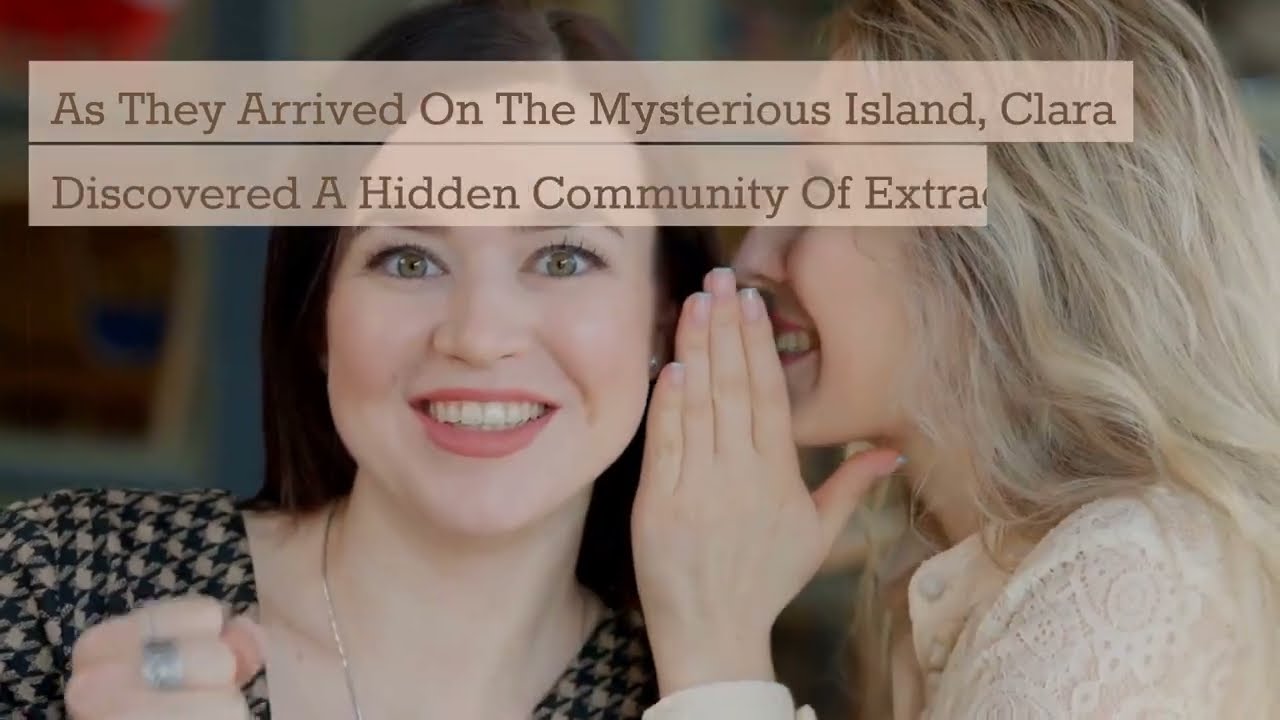The color photograph captures a humorous and intriguing moment between two women. The woman on the left, with long, straight black hair parted on the left, hazel eyes wide open, and a frozen smile, appears to be listening intently. She has fair skin, berry-colored lipstick, and is wearing a black top with a white pattern, complemented by a silver chain necklace. Her right hand, adorned with a silver ring, is raised to shoulder height, clenched in a fist suggestive of anticipation or excitement. Facing her at a 90-degree angle, the woman on the right has long blonde hair and is wearing an intricate, lacy white blouse. With her left hand held up next to her mouth, she seems to be whispering a secret, smiling broadly as she does so. 

In the background, a brown picture frame with a reddish image can be faintly seen. Overlaid at the top of the image in light brown, semi-transparent boxes with dark brown text, the words read: “As they arrived on the mysterious island, Clara discovered a hidden community of extra…,” with the last word cut off, adding an element of mystery to the scene. The overall setting is enriched by the medium brown background that ties the composition together.